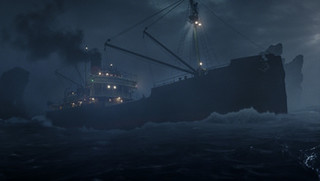The image appears to depict an illustrated, dark nighttime scene of a large cargo ship or barge traveling across a cold, dark ocean. The vessel is moving from left to right amidst rippling waves that splash against its hull, creating white foam at the bow. Dominating the forefront of the ship is a prominent black smokestack emitting thick, dark smoke into the dreary night sky, which is dotted with scattered clouds and possibly faint stars. The ship’s superstructure is white and illuminated with numerous lights, creating a stark contrast against the surrounding darkness. Multiple cranes and booms, tethered with ropes, extend from the central part of the ship in a V shape, seemingly assisting in the ship's operations. The vessel spans several stories high, each deck lined with lights. Despite the clarity of the ship's upper features, the overall scene is quite dark, making it hard to discern further details in the background, although there might be additional hulls or even cliffs and glaciers emerging from the water.